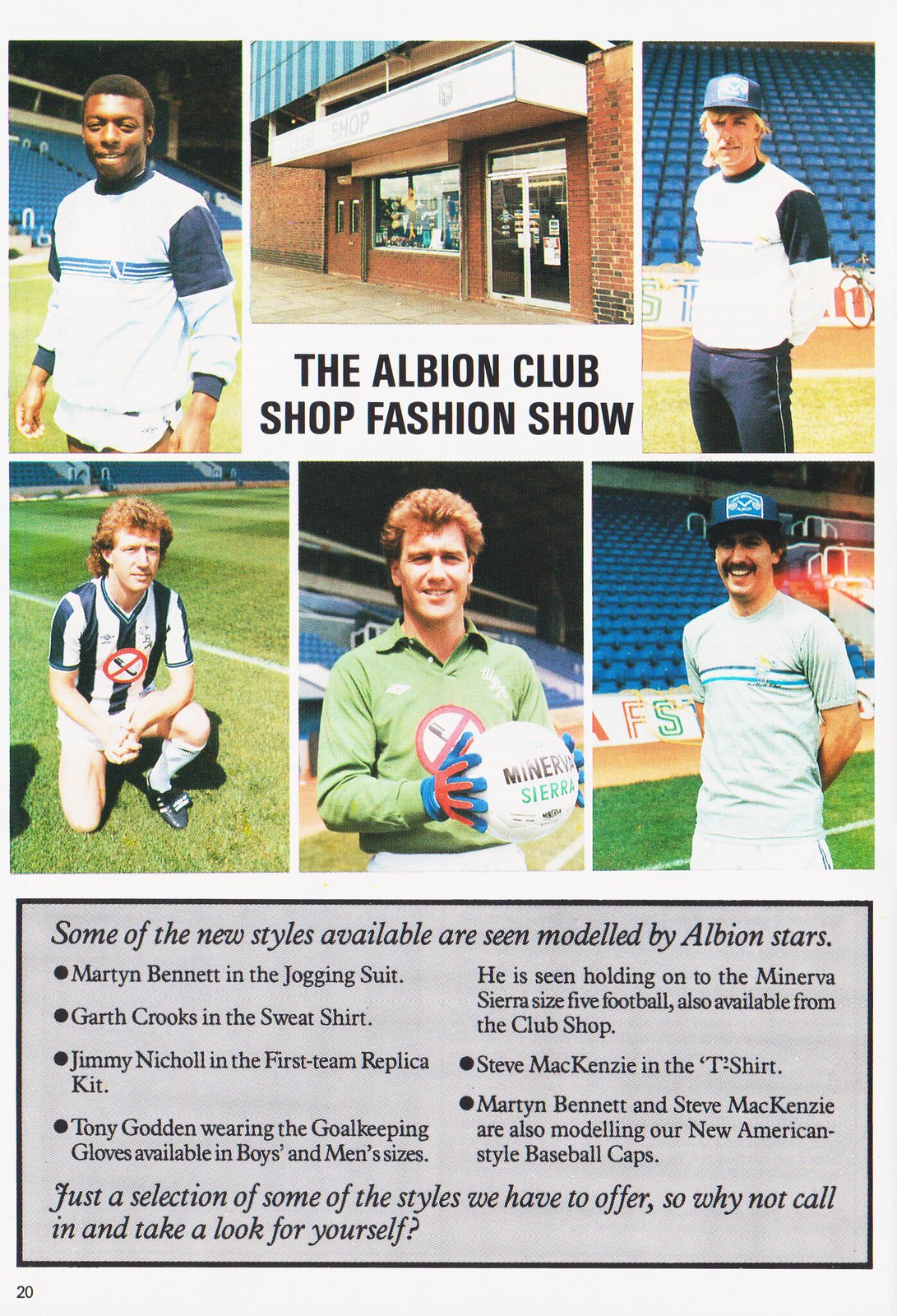The image displays a magazine page or flyer with a white background, featuring six rectangular photos arranged in two rows of three. Each rectangle contains an image of male athletes modeling apparel against the backdrop of a soccer field or stadium. 

In the top row:
- The first image shows an African-American male in a white and blue soccer uniform, standing on a soccer field.
- The second image features the front of a building with the caption "Albion Club Shop Fashion Show".
- The third image depicts a white man with blonde hair wearing a blue cap, white sweater, and blue pants, in front of a soccer stadium.

In the bottom row:
- The first image shows a white man with goldish-brown hair kneeling on grass in a striped black and white soccer uniform.
- The second image displays a man with goldish-brown hair in a green shirt and red and blue gloves, wearing white pants, likely a goaltender, posing with a soccer ball.
- The third image includes a white man with a mustache, a blue cap, white shirt, and white pants, with a soccer stadium backdrop.

Below these rectangles is a gray box with a black border, featuring black text that reads: "Some of the new styles available are seen modeled by Albion Stars." This section lists:
- Martin Bennett in a jogging suit.
- Garth Crooks in a sweatshirt.
- Jimmy Nichol in the First Team replica kit.
- Tony Giddens wearing goalkeeping gloves, available in boys' and men's sizes, holding the Minerva Sierra size 5 football, also from the club shop.
- Steve McKenzie in a t-shirt.
- Martin Bennett and Steve McKenzie also modeling new American-style baseball caps.

The text concludes: "Just a selection of some of the styles we have to offer, so why not call in and take a look for yourself?" The bottom left corner indicates "20", signifying the 20th page.